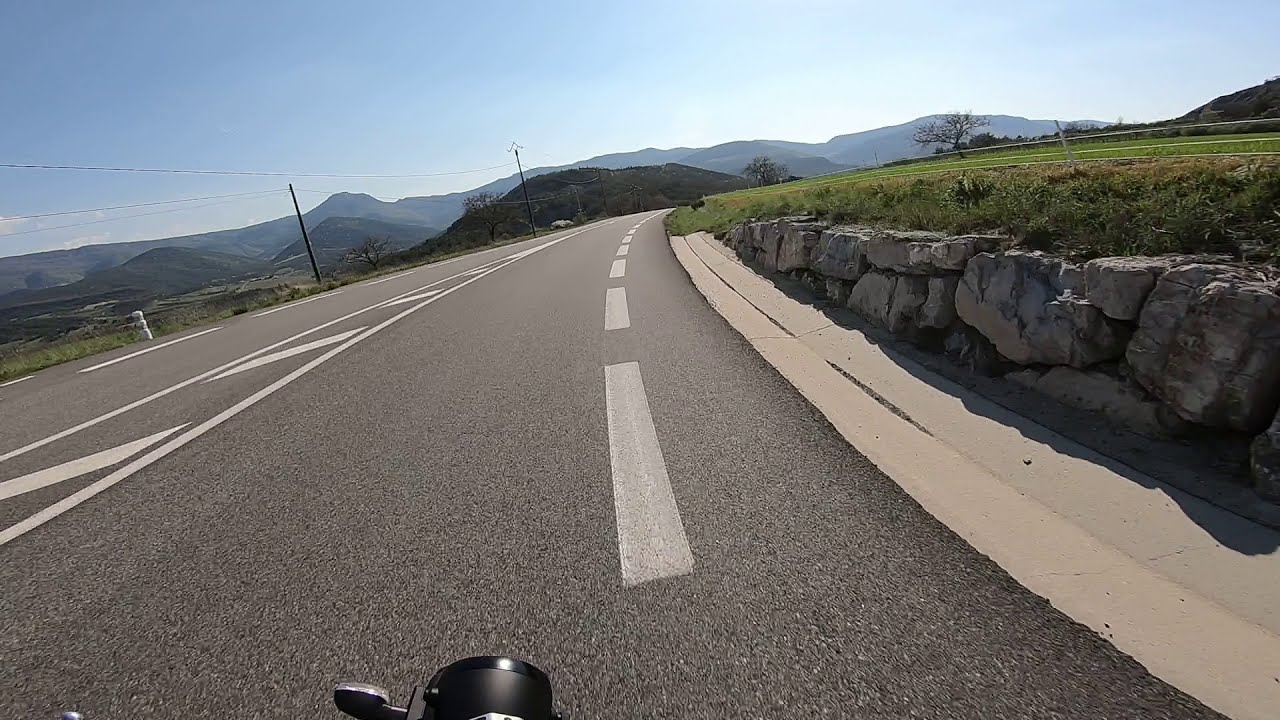This image captures the perspective of someone riding a motorcycle on a multi-lane highway during the middle of the day, framed within a horizontal rectangle. The road, primarily gray with distinct white markings, stretches from the bottom center and curves slightly to the right. The white lines, both dashed and diagonal, guide the flow of traffic, with additional vertical white blocks marking the road edges.

On the right side, a rock wall supports a bank of vivid green grass, and we see several utility poles with power lines. On the left side, the landscape features rolling hills and mountains in hues of dark brown and tan. The sky above is a clear, light blue, indicating pleasant weather. The overall scene is a mix of man-made roadway and natural, green surroundings, highlighting a picturesque ride through this highway setting.